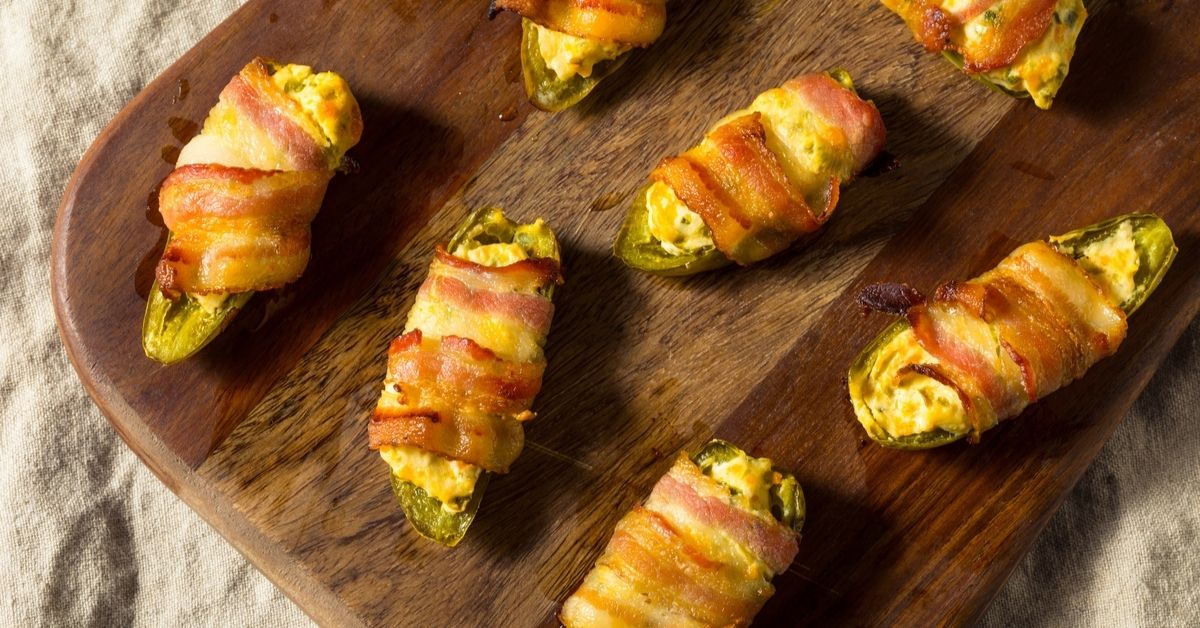This image captures a delicious appetizer of jalapenos stuffed with a yellow cheese and wrapped in crispy bacon, neatly arranged on a rectangular wooden cutting board with rounded edges. The cutting board sits on a wrinkled, tan canvas-like tablecloth, enhancing the rustic presentation. The jalapenos, cut in half and slightly blackened from baking, display an inviting combination of colors: the green of the peppers, the golden hue of melted cheese oozing out, and the appetizingly browned bacon, crispy from the oven. The photograph, with a rectangular aspect ratio (twice as long on the top and bottom as on the sides), showcases seven of these savory treats, glistening with bacon grease and exuding a mouthwatering appeal.